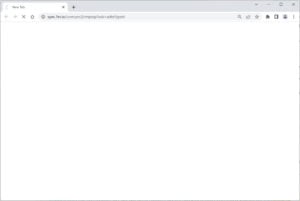This image depicts a desktop computer screen with a blank browser window that appears to be loading. On the top of the screen, there is a white tab with a loading circle to the left, indicating that the page is in the process of loading. To the right of this tab is a plus sign, used for opening a new tab. In the header section of the browser, there are several icons: a plus sign, a minus sign, an X, a refresh button, and a house icon which signifies the home button, although its details are a bit unclear. Additionally, there is a website address bar present. To the right of this address bar, there is a magnifying glass icon for searching, followed by another small symbol that is hard to make out due to its size. Next to it, there is a star icon for bookmarking, a puzzle piece icon representing plugins, a square icon, a profile icon, and three vertical dots indicating a menu. The overall outline and the icons are in gray, giving the interface a minimalistic appearance.